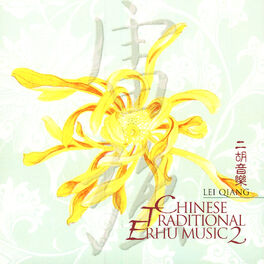The image depicts a square album cover set against a pale seafoam green and white background. The central focus is a vivid yellow chrysanthemum, with long, windblown petals painted in shades of gold and orange. Beneath the yellow flower is a layer of Chinese calligraphy characters in a light gray tone, which extends vertically across the center of the image. To the right side of the cover, more Chinese text is stacked, and directly beneath it, in smaller English text, it reads “Lei Qiang” (spelled L-E-I Q-I-A-N-G). The album's title appears in darker red capital letters near the bottom right corner: "Chinese Traditional Erhu Music 2," emphasizing it as the second volume of a collection. The background's soft teal hues, coupled with the gentle, watercolor painting style, evoke a calming and serene aesthetic, making the vibrant yellow chrysanthemum stand out prominently against the muted backdrop.